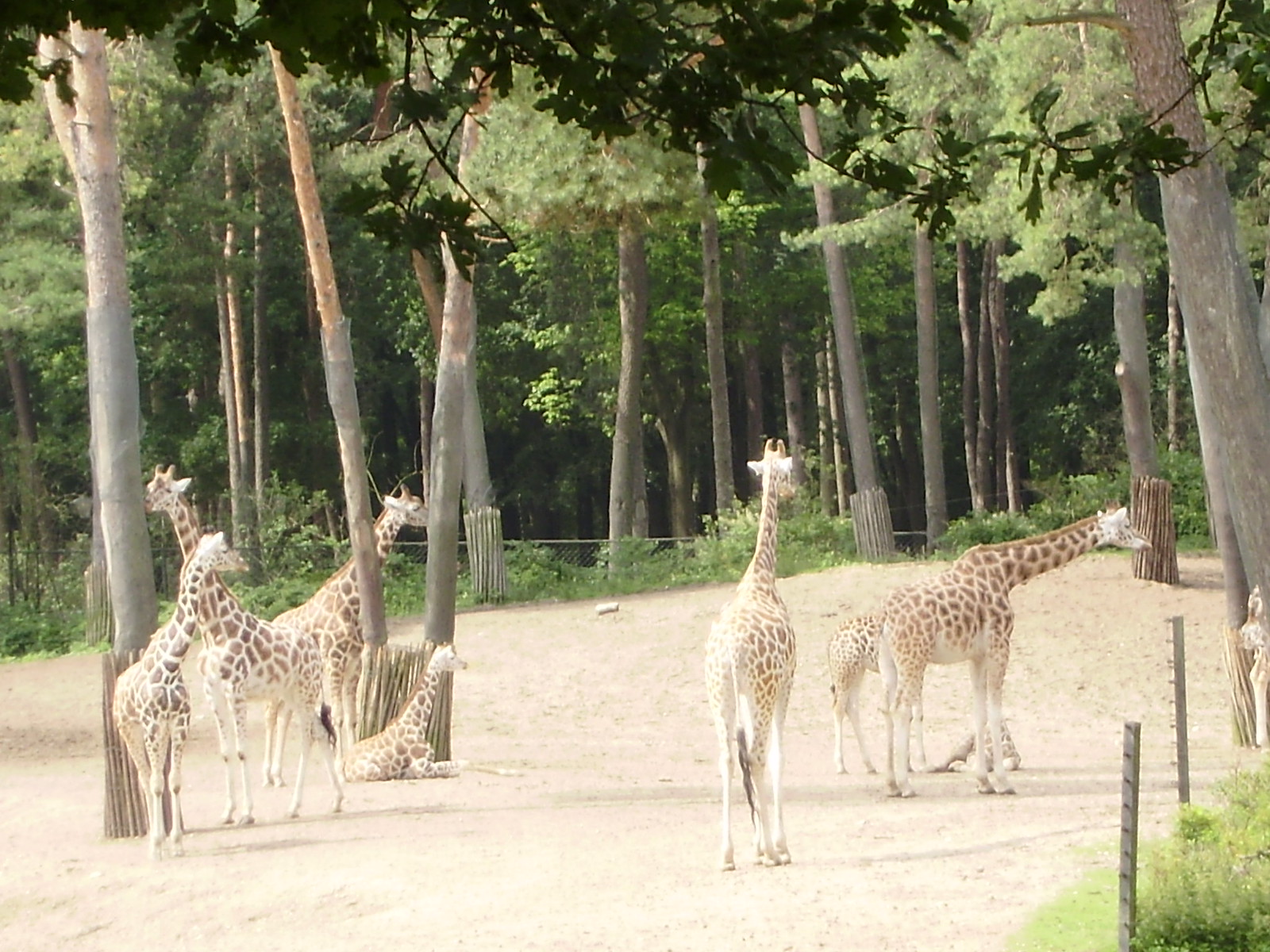The photograph depicts an exhibit at a zoo featuring eight giraffes of varying sizes and ages, with five adults and three calves. The enclosure has a sandy, dry ground surface and is surrounded by a fence made of metal poles and thin wiring, which might be electrified. Within the enclosure are several tall trees, many with wooden protectors around their bases to prevent the giraffes from damaging them, though some bark has clearly been stripped away. The backdrop of the exhibit reveals a dense, dark forest with gray tree trunks and lush green foliage, contrasting with the brighter, somewhat overexposed foreground. The giraffes are positioned in two main groups: one group of four on the left, where three are standing and one is sitting, and a group of three on the right, dominated by a large adult, possibly a mother, with a calf partially obscured behind her, showing only its back end and legs. The only visible part of an eighth giraffe is its leg, just off the right edge of the image.